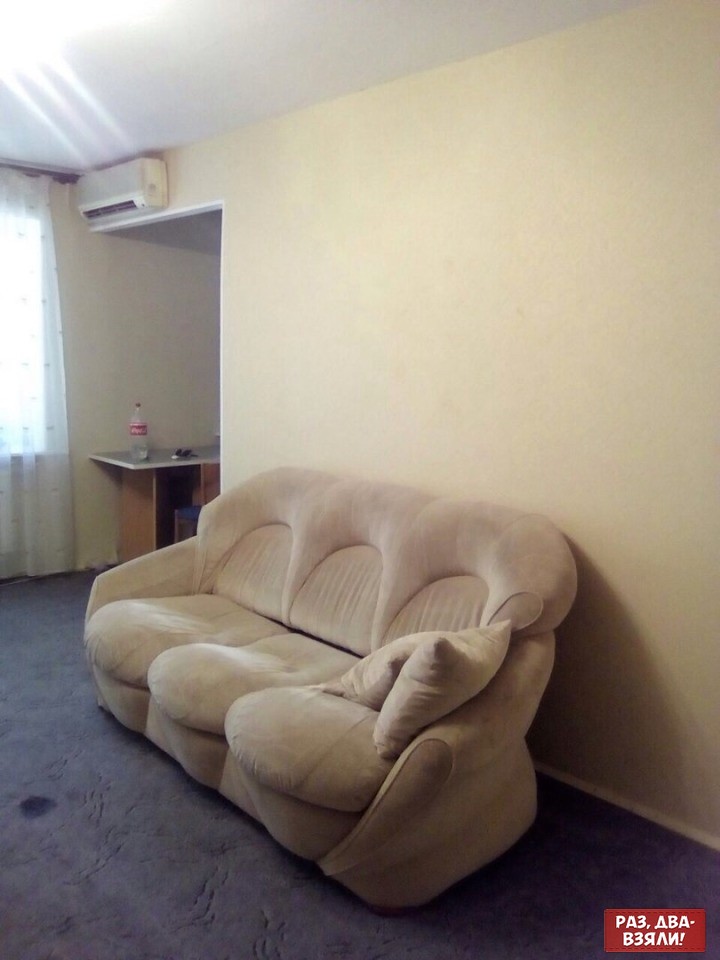The photograph captures a living room with a grey, patterned carpet and walls painted a custardy yellow leading up to a white ceiling. The focus of the image is a large, plush, cream-colored couch at the center, equipped with two pillows on its right side. To the left, light filters in through a window covered by a white curtain. An air conditioning unit is visible above a doorway in the upper left part of the image, leading to a hallway. Below the air conditioner, a small table holding what appears to be an empty bottle of Coke is tucked against the wall. The overall ambiance of the room is bright, likely due to natural daylight or an overhead light source.